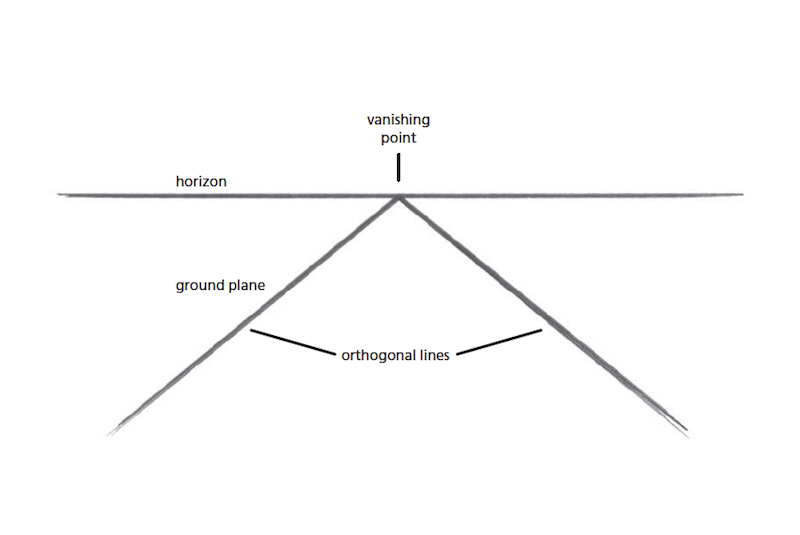This black and white sketch illustrates the artistic concept of a vanishing point. Central to the image is a horizontal line labeled "horizon," running from left to right. At the very center of this horizon line is a point marked as the "vanishing point." From the bottom left and bottom right of the diagram, two angled lines converge upward, meeting precisely at this vanishing point. These angled lines are identified as "orthogonal lines." The area between them, below the horizon line, is labeled "ground plane." The overall composition gives the illusion of looking down a road, demonstrating how lines appear to converge at a point on the horizon in perspective drawing, which is a fundamental principle in optics and imaging.